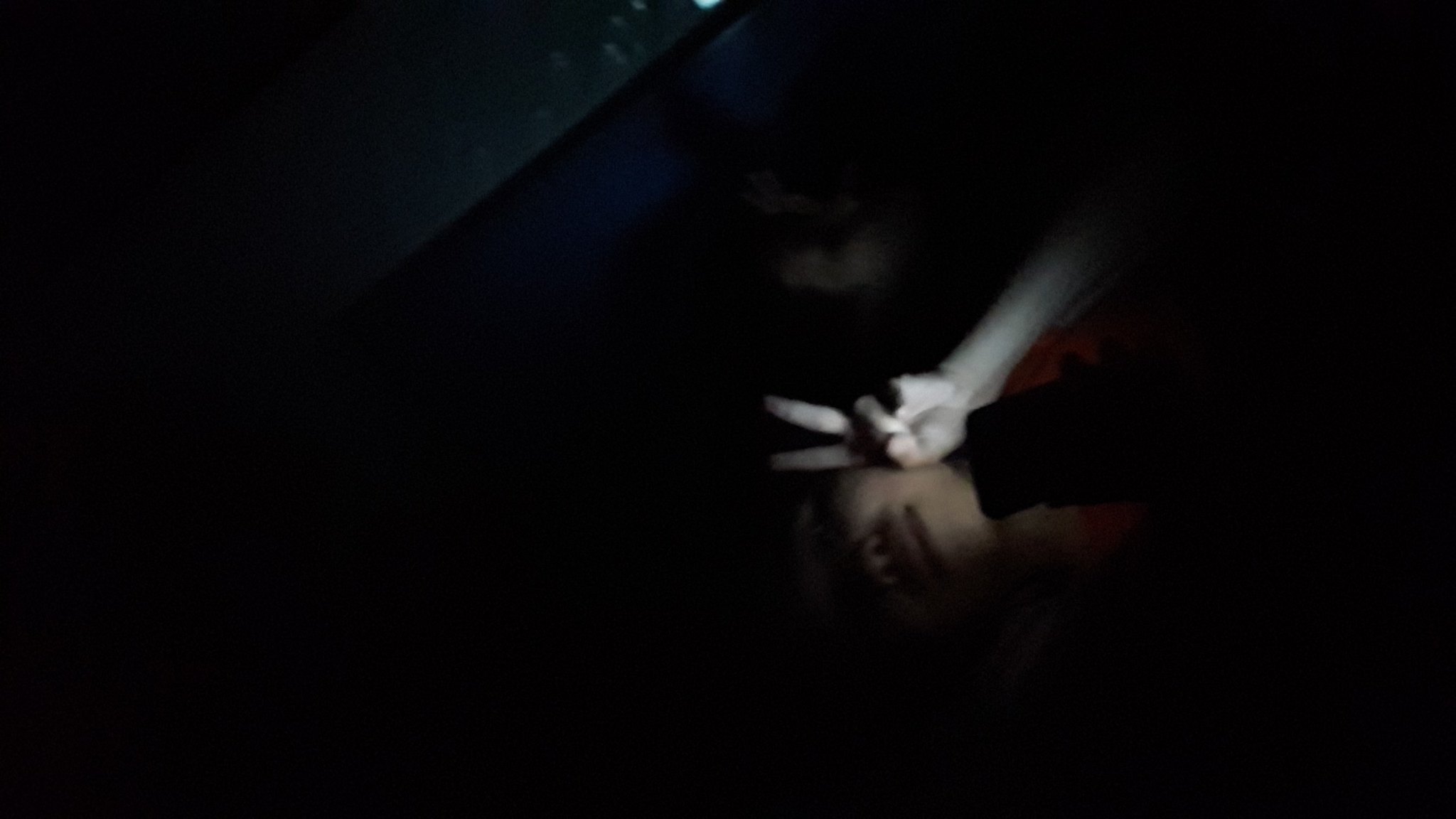Against a stark black background, a barely illuminated individual holds up a peace sign close to their face. The person has their index and middle fingers extended while their thumb, ring, and pinky fingers are curled inward. Their facial expression is characterized by pursed lips, forming a subtle "duck face." The dim lighting reveals just a glimpse of their neck, hinting at the contours of their body, which fades into the darkness. The overall mood of the image is mysterious and understated, with the person partially obscured by shadow.